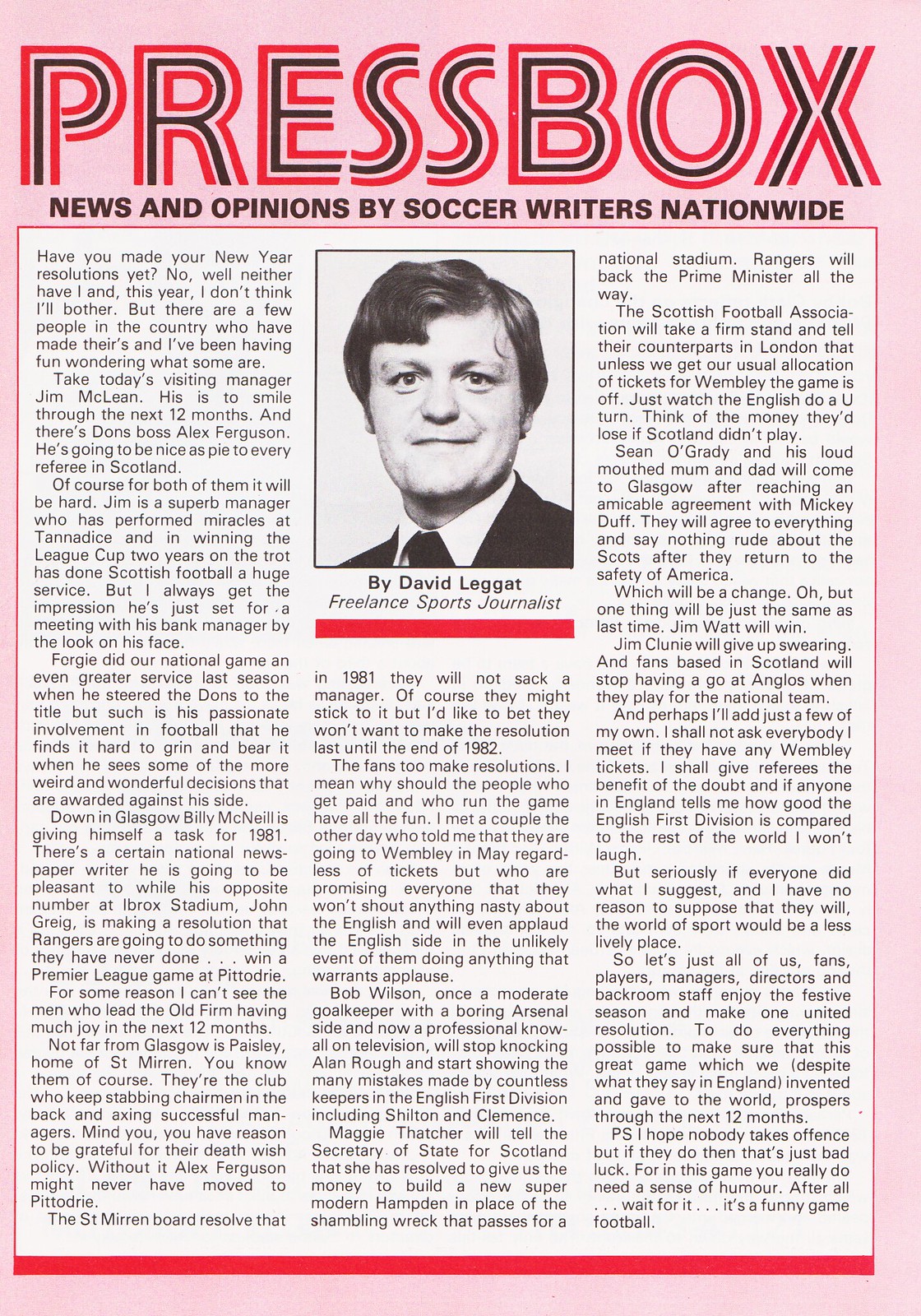The image depicts a page from what seems to be a magazine or soccer program, dated around 1981. The background is a pale pink, featuring a prominent headline at the top that reads "PRESS BOX" in a striking combination of red and black capitals. Beneath the headline, in bold black capitals, it states, "NEWS AND OPINIONS BY SOCCER WRITERS NATIONWIDE." The article is structured in three columns, with a headshot of a man, identified as David Leggett, a freelance sports journalist, at the top of the middle column. David Leggett, a clean-shaven white man in a suit jacket, white dress shirt, and tie, gazes directly at the camera. The page also includes red underscores, both below David's name and at the bottom of the page, emphasizing part of the layout. The text is dense with news and opinions concerning soccer, referencing the years 1981 and 1982 multiple times.